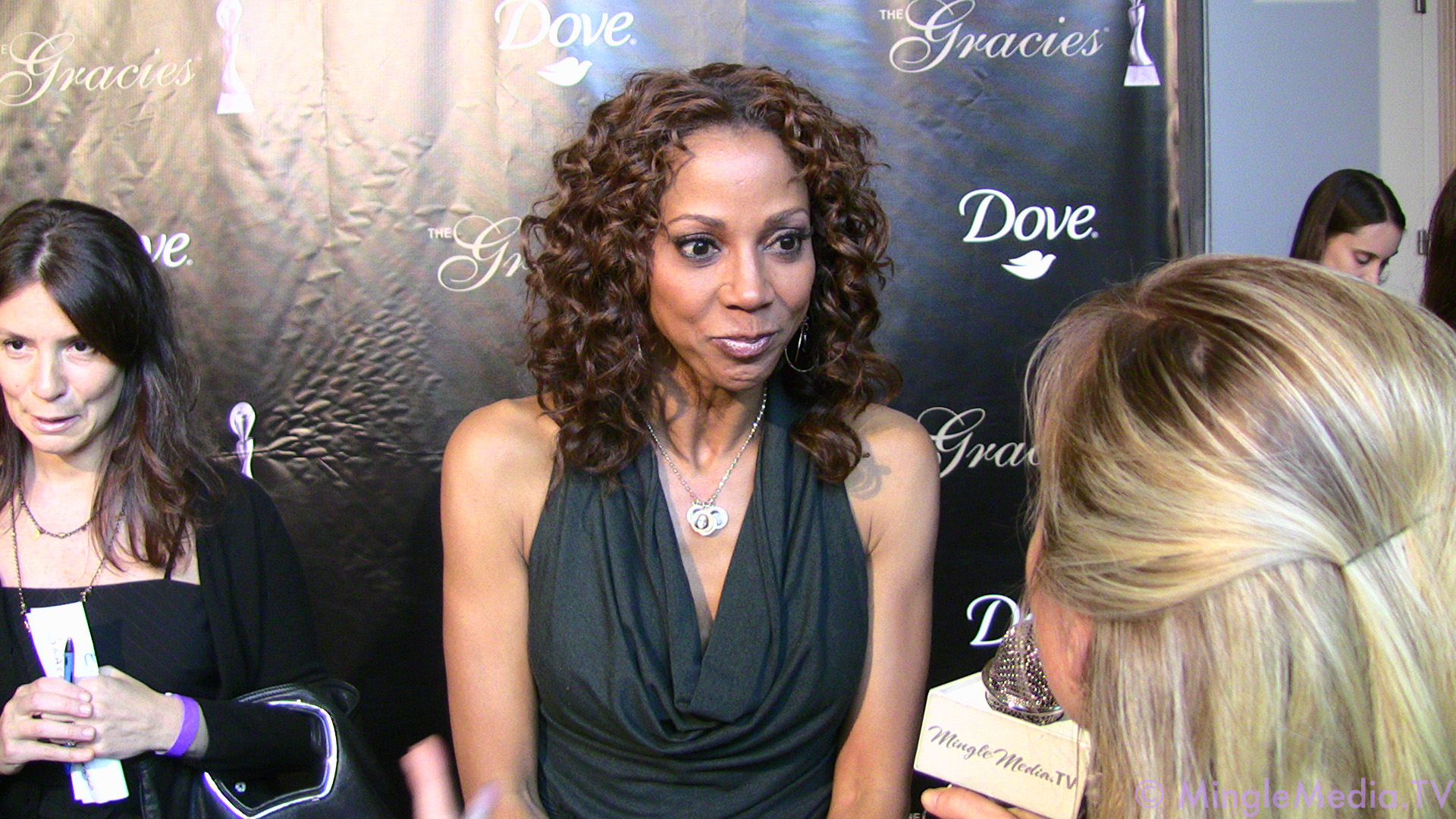In the photograph, a woman stands in the center, giving an interview. She has curly brown hair framing her face and dark brown eyes. Her lips are pursed slightly, suggesting she is about to speak or smile. She is adorned in a sleeveless, black evening gown with a low neckline, which gathers in a stylish v-neck. Around her neck, she wears a silver chain necklace with an oval pendant, complemented by silver hoop earrings. Her gaze is directed towards the bottom right corner of the image, where the back of the interviewer’s head is visible. The interviewer, with blonde hair, is holding a shiny black microphone encased in a white box bearing the text "Magic Media TV" in black letters. In the lower left corner of the image, another woman with long brown hair and a black outfit is standing, holding a pen and paper. The backdrop behind them is black with multiple white logos that read "The Gracies," accompanied by the word "Dove" and an outline of a bird in profile beneath it.